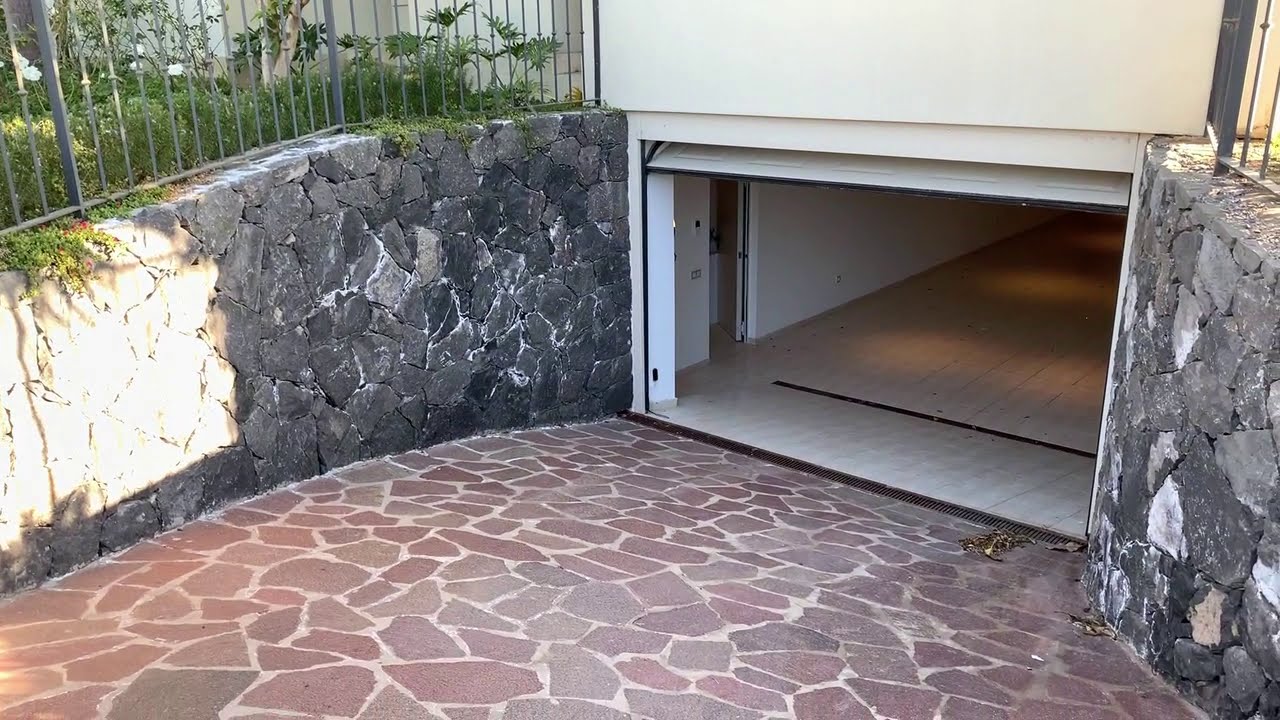The image depicts a detailed view of a stone-paved driveway leading down to an underground garage. The driveway features rocks in varying shapes and sizes, with colors ranging from light red and burgundy to light black, and it is bound with white mortar. On each side, there are dark gray, charcoal, and black rocky walls, and running along these walls are gray metal fences.

As the driveway descends, the walls become higher, creating a more enclosed feel as it approaches the garage. The garage door is open, revealing a light tan, tile floor inside. A strip resembling a grate is visible a few feet into the garage, likely for water drainage. Inside the garage, to the left, there is an open "man door" that provides access to the interior of the home. Above the garage, the lower portion of a white building is visible, hinting at the structure situated above. Additionally, some green plants can be seen growing behind the left-side gray fence. 

The entire scene is illuminated, with the garage lights adding a touch of brightness to the otherwise stone-heavy and somewhat somber environment.